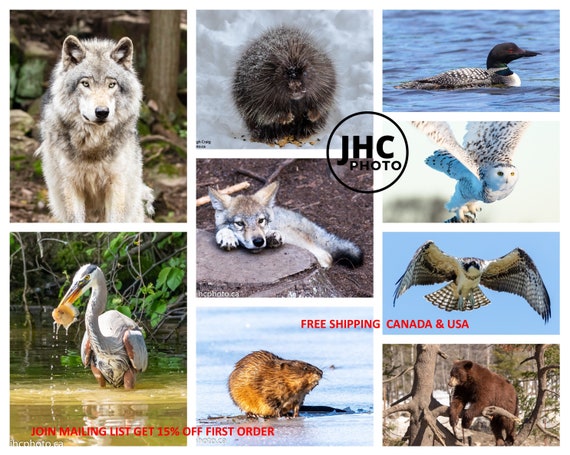The image is a collage of vibrant wildlife photos, marked by a JHC Photo logo offering "Free Shipping Canada and USA" and a 15% discount for joining their mailing list. The collage is organized with four images vertically on the right, three in the center, and two on the left. At the top left, a wolf stands against a natural backdrop. Below, a portrait of a porcupine and a mallard duck swimming are prominently featured. The center column includes a magnificent snowy owl in flight, a hawk soaring, and a bear—likely a brown bear—reaching over a branch. The bottom right showcases an otter vigorously shaking off water. Additional details feature a fisher bird standing and hunting in water, and a pelican catching something with its beak. Among other creatures, we see a coyote or wolf, a small groundhog-like animal, and another fox. The scene is rich with wildlife, capturing the essence of Canadian and Alaskan nature.